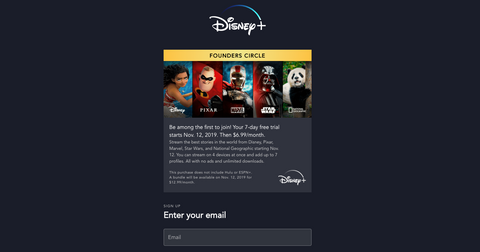The image appears to be a screenshot of the Disney+ welcome or sign-in page. At the top, there is a blank background where "Disney+" is prominently displayed. Below this, a yellow banner is featured at the top of a box that reads "Founders Circle." 

Beneath the banner, there are five images arranged side-by-side representing various Disney+ content categories: Disney, Pixar, Marvel, Star Wars, and National Geographic. Under these images is a passage written in white text on a gray background. The Disney+ logo is situated in the bottom right corner of this gray section.

Further down, there is another section prompting users to "Enter your email" in white text, accompanied by a gray field where the email can be input. The background of this lower part of the page is black.